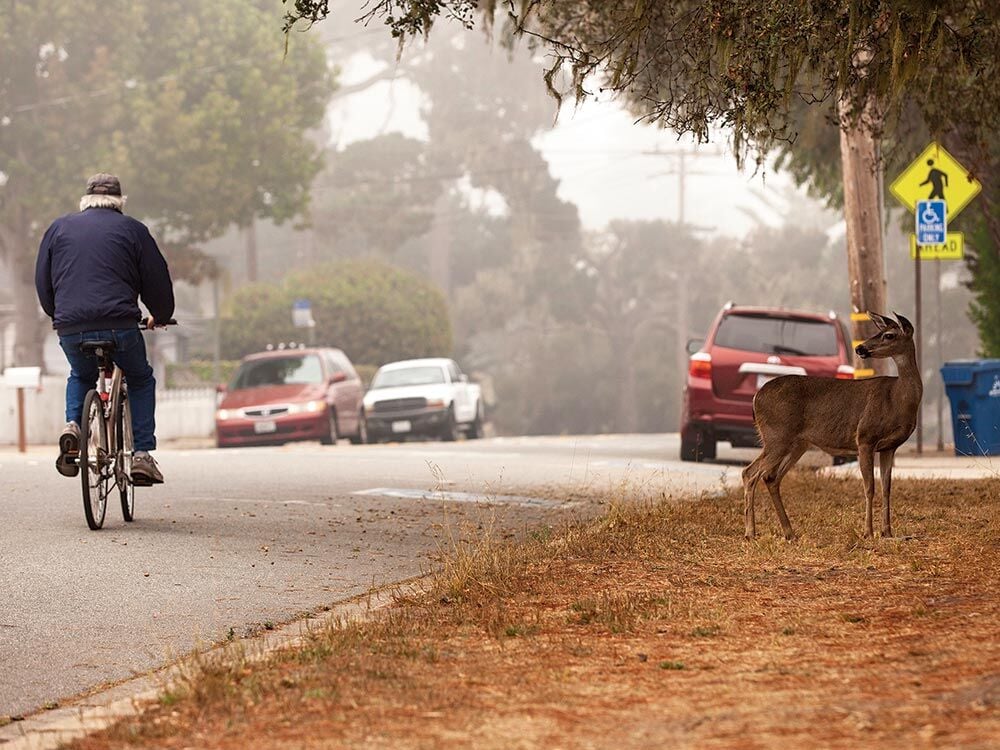In this outdoor scene, set in what appears to be a small town or neighborhood, a man with gray hair rides a bicycle away from the camera. He wears a navy blue jacket, blue jeans, sneakers, and a ball cap, and pedals down the road. Three cars are parked on either side of the street: a red vehicle on the right, and a white truck and red van near a white picket fence on the left. The sky is overcast and hazy, with large trees, power lines, blue trash cans, and street signs complementing the background. On the right side of the image, a small, not fully grown deer stands on a dirt sidewalk with some weeds and dried brown grass, looking back at the man. A white mailbox on a brown wooden post is also visible. The juxtaposition of the man focused on the road and the deer gazing at him adds a quirky touch to the scene.